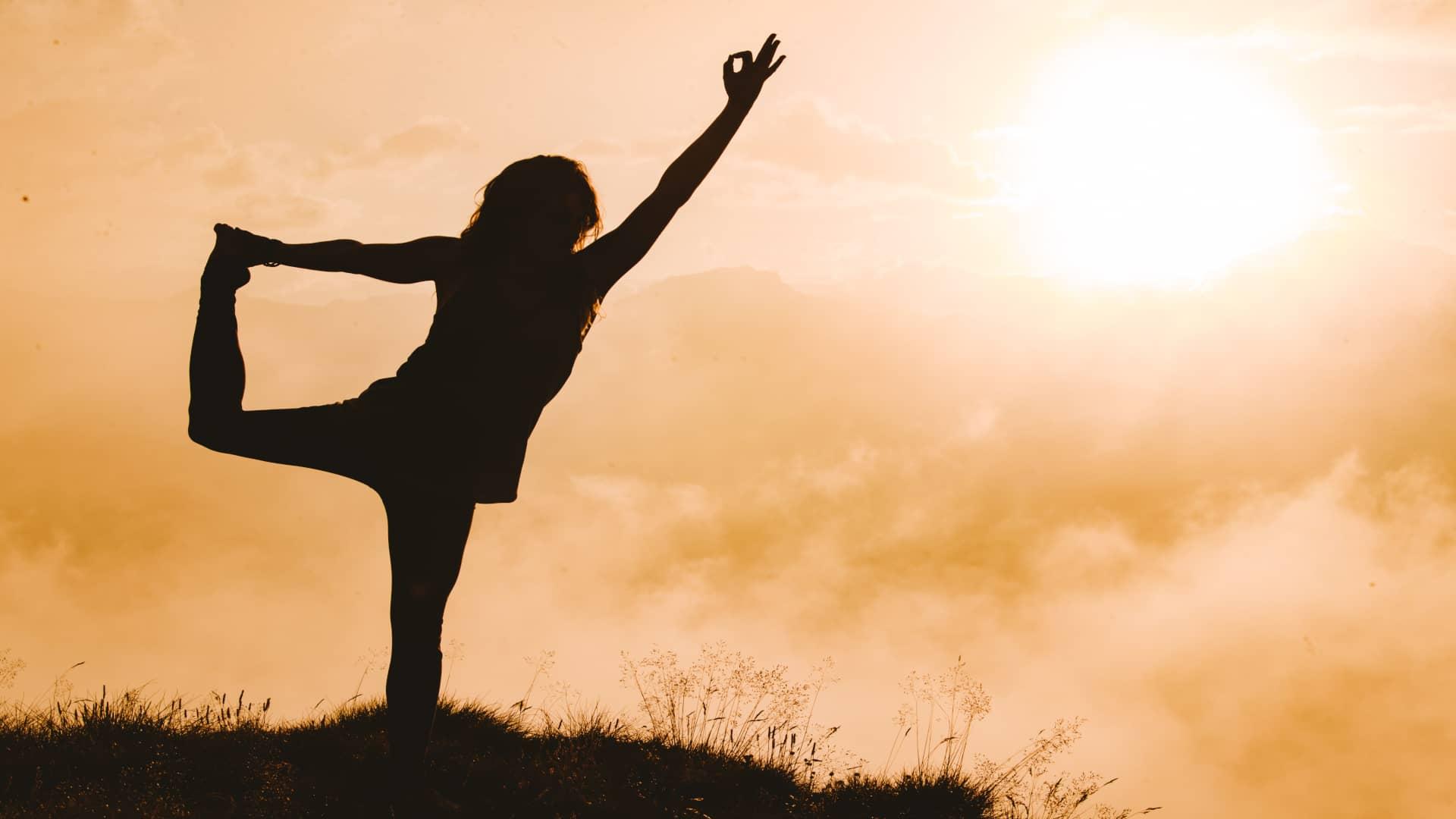The photograph captures a striking scene at golden hour, with the warm hues of a setting sun casting an orangey-yellow glow across the sky filled with wispy clouds. In the foreground stands a silhouetted figure on a grassy hill, the texture of the grass detailed against the vibrant backdrop. The figure, likely a woman identified by her long hair and form-fitting outfit, is gracefully performing a yoga pose. She stands balanced on one leg, with her other leg bent behind and held by her outstretched hand. Her free arm reaches up towards the sky, her fingers forming an 'okay' sign. The overall effect is a serene and striking image, blending the warm tones of the sunset with the graceful, dark outline of the woman in her pose.